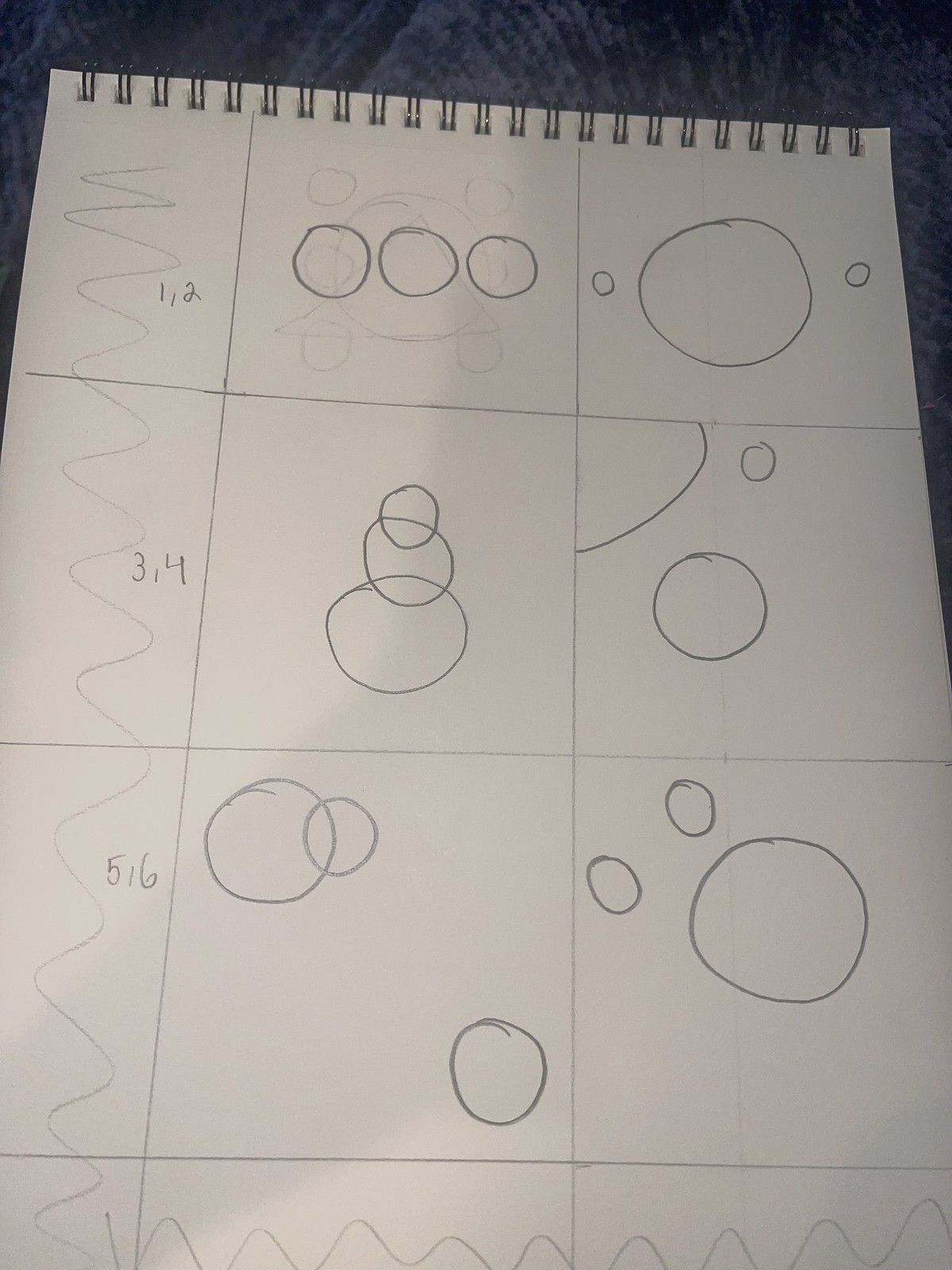The image depicts a detailed drawing on a notebook page with a black and gray countertop background. The notebook is identifiable by the small metal rings on the top edge, securing the white page. The page is segmented into seven distinct squares arranged in two rows. 

- The **first square** contains the notation "1, 2" accompanied by a squiggly line and three circles.
- The **second square** features a large central circle flanked by two smaller circles.
- The **third square**, situated on the second row, is labeled "3, 4" with a squiggly line crossing through it, and three touching circles.
- The **fourth square** showcases a whole circle, a half-circle positioned in the corner, and one small circle.
- The **fifth square** holds the label "5, 6" with another squiggly line and remains otherwise unelaborated in the voice description.
- The **sixth square** presents a large circle interconnected with a smaller circle, and a solitary circle is placed at the bottom right corner.
- The **seventh square** features a large circle encompassing two smaller interior circles.

At the bottom of the page, three small pieces of squares with squiggly lines through them are noted. The composition suggests a structured pattern or perhaps a constellation of various graphical symbols and mathematical annotations.